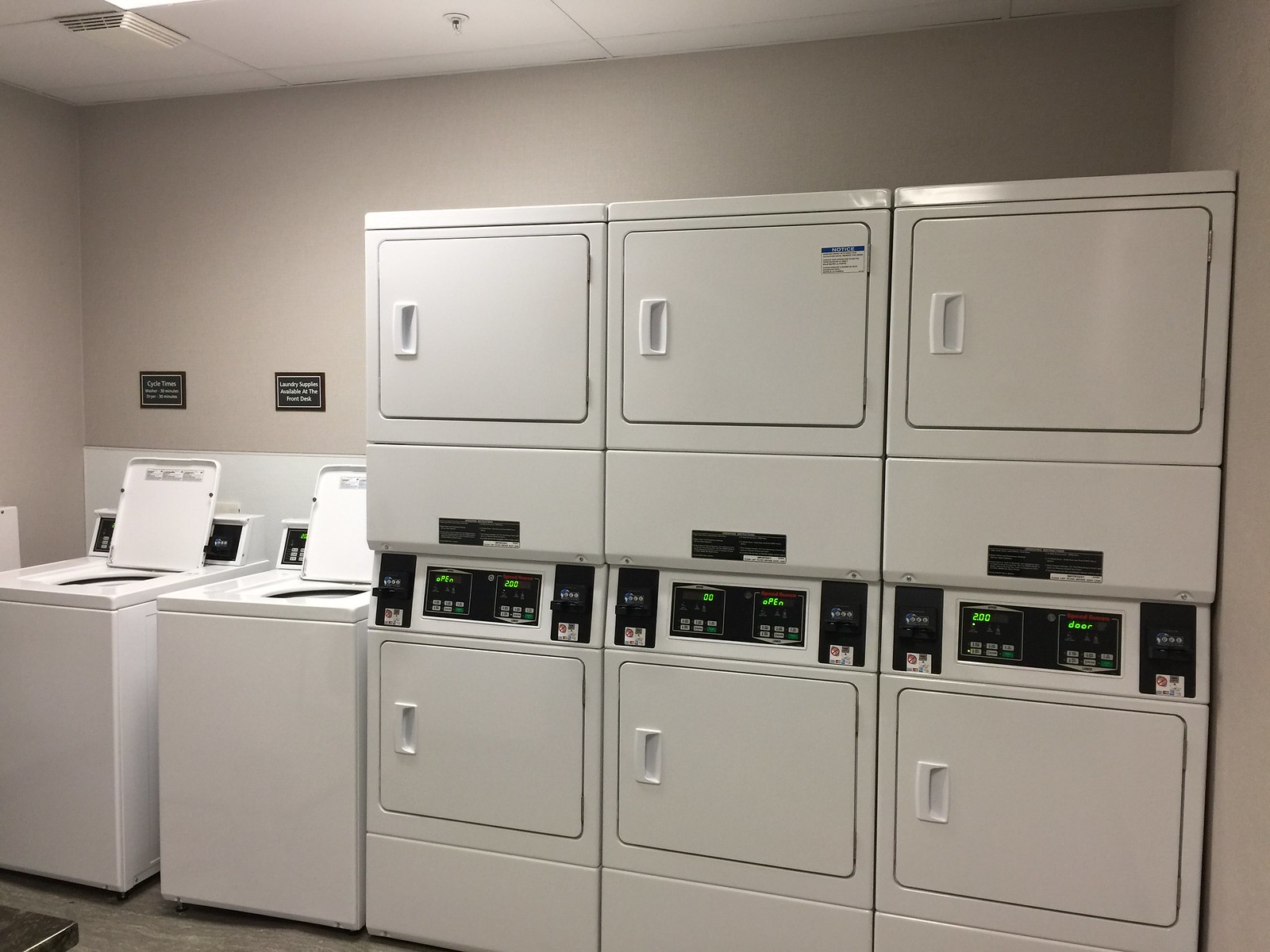The image depicts a typical laundry room in an apartment complex, featuring a lineup of laundry equipment. Positioned against a very light beige wall, the scene includes two top-loading washing machines on the left-hand side of the image, with their lids open, facing slightly to the left. Beside these washers, there are six front-loading dryers, stacked in sets of three. These dryers have coin-operated mechanisms located between the top and bottom units and display screens showing the remaining time. The washers and dryers are all a standard white color. 

Above the washers, there is a black sign with white lettering, and small signs with similar style can also be seen above the dryers, likely containing operational instructions. The ceiling is bright white, contributing to the room's modest lighting, and the flooring appears to be a grey vinyl. The dryers feature green lights indicating their operational status, and their front-facing doors are all basic square designs. Overall, it's a functional and straightforward laundromat setup within the apartment complex.